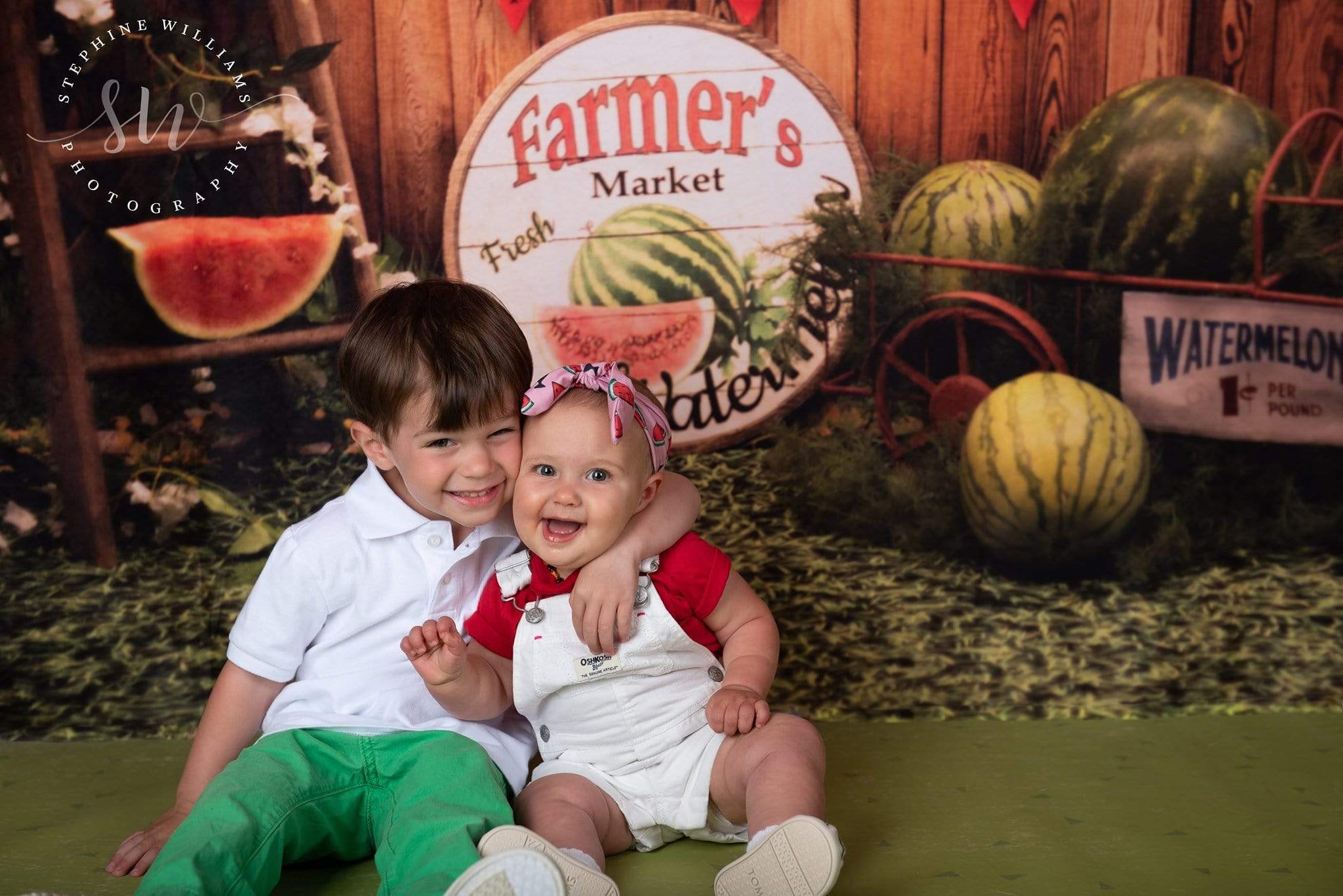In this professional photograph by Stephanie Williams Photography, two children are the focus. A little boy, approximately three years old, with dark brown hair and a beaming smile, is dressed in a white button shirt and bright green pants. He lovingly hugs his baby sister with his left arm. The infant girl, adorned with a pink headband decorated with watermelon slices, matches her brother’s cheerful expression. She wears white Oshkosh overalls and a red shirt, and has a delightful set of white shoes on her little feet.

The setting mimics a rustic farmers market. A wooden backdrop is embellished with a large, round sign painted white that reads “Farmers Market Fresh” in red and black, featuring a depiction of a striped whole watermelon and a juicy, red watermelon slice. To the left, a wooden ladder holds another slice of watermelon, while silk white flowers and green leaves add to the aesthetic. On the right, an old-fashioned red metal wagon is filled with watermelons and displays a sign that reads "Watermelon 1¢ per pound." The children sit on a green carpet that resembles grass, adding an extra touch of authenticity to the market scene. This charming and meticulously arranged photograph captures the innocence and joy of childhood against a beautifully crafted backdrop.